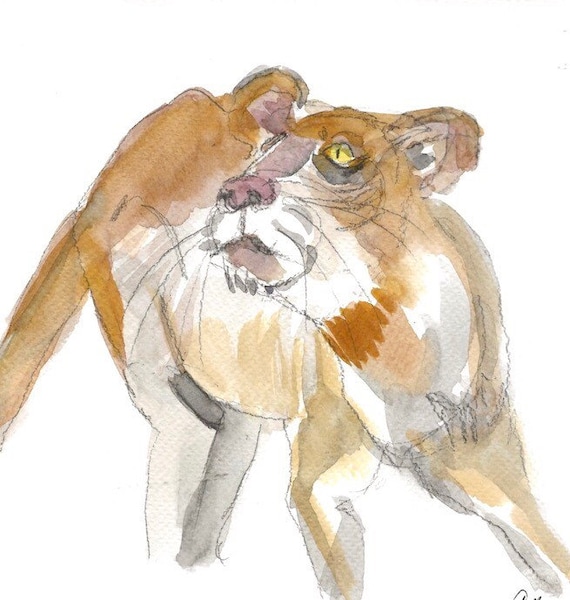This watercolor artwork depicts a wildcat, likely a female lion or cougar, showcasing its intricate details. The wildcat stands in motion, with its head turned left, capturing the dynamic shift from right to left. Its body is mostly a tawny, light brown color reminiscent of coffee with creamer, transitioning to darker brown and gray shades toward the legs, with a noticeable amount of shading under the mouth. 

Its large, round, light brown ears and distinct, pale pinkish-purple nose add to its lifelike appearance. The wildcat’s bright yellow eyes with narrow black slits draw immediate attention. Long, black whiskers sprout from the mouth area, with four on each side, accentuating the face. Meanwhile, the legs—three of which are visible—extend downwards, showing their bending motion, and a long tail trails behind, partially disappearing out of the frame. The softness of the watercolor technique is evident, with colors blending smoothly without sharp edges.